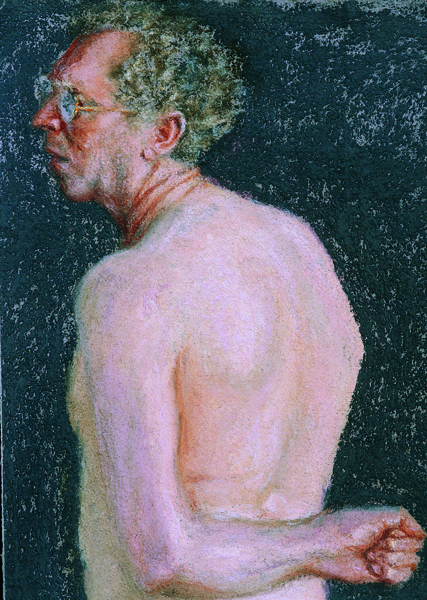This is a vertical rectangular painting of an older, partially nude man viewed from the back and waist up. His exposed skin is a light beige, contrasted by his somewhat darker, ruddy face. The background features a dark, almost charcoal-gray hue with subtle blue and white smudges. The man is facing left, with his left arm bent behind his back, his fist clenched near his spine. He has short, curly gray hair and a receding hairline, wearing wire-rimmed glasses on his notably reddish, somewhat stubbly face. His shoulders are slightly stooped, and delicate black lines add texture to his otherwise pale back, emphasizing his age and weariness. The overall composition highlights his vulnerable, stooped posture against a stark, moody backdrop.